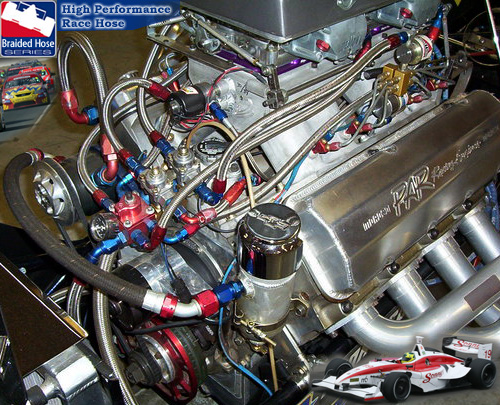This image prominently features a high-performance race car engine, spotlighting its intricate design as part of a braided hose series advertisement. Dominating the image is a large, stainless steel motor adorned with various red and blue hoses, and numerous wires and pipes, all converging to form a complex and sophisticated system. The engine gleams with a chrome or silver finish, amplifying its high-quality construction. Centered on the motor is the brand name "PAR," underscoring the product’s identity. Above the engine, the text "Braided Hose Series" in blue font alongside "High-Performance Race Hose" is displayed, featuring an emblem in red and blue. Supplementing the mechanical focus, the bottom right of the image showcases a red and white Formula One race car, juxtaposed with NASCAR vehicles situated in the background, collectively emphasizing the race-proven reliability and performance of the advertised hoses.